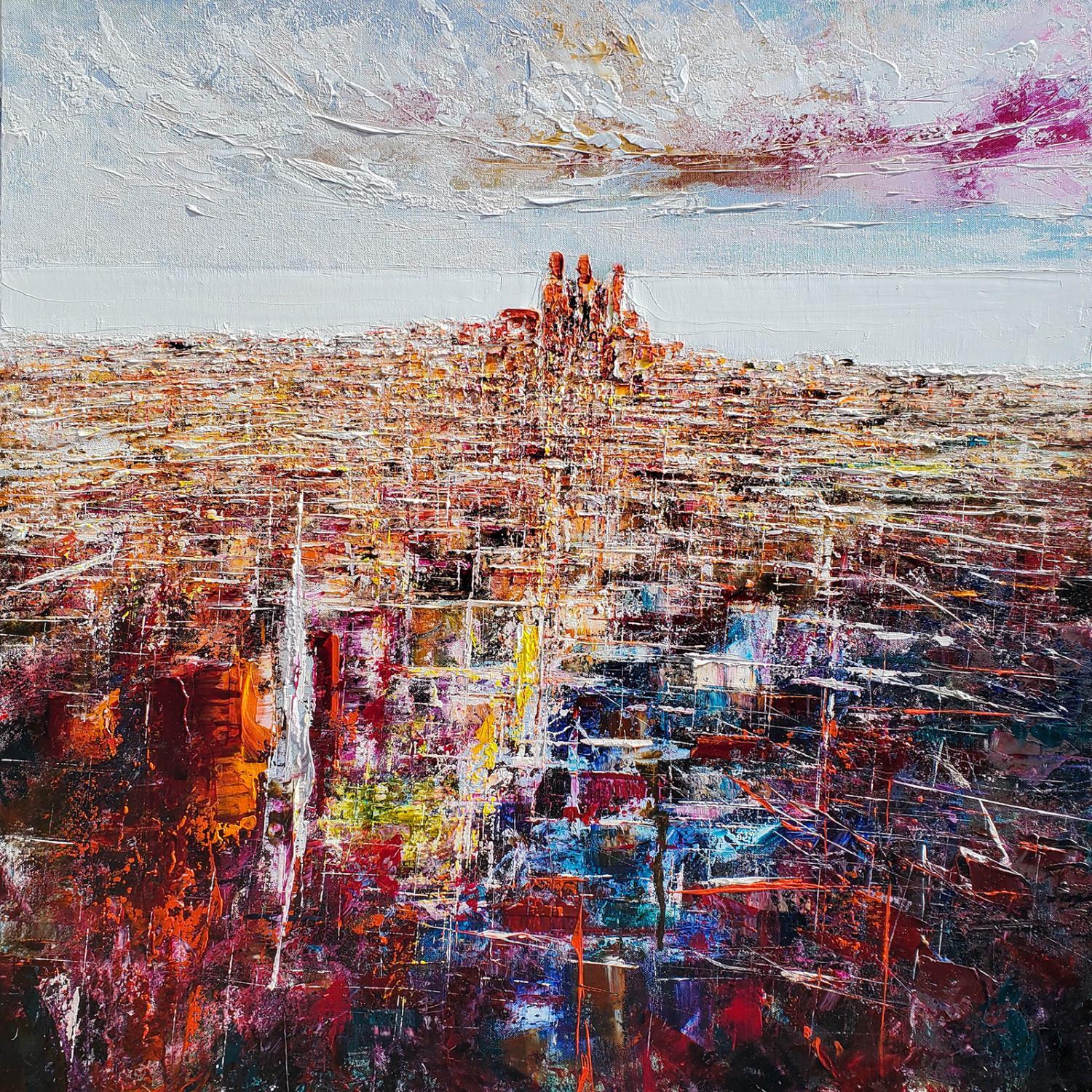The image depicts an abstract, textured landscape that evokes the semblance of a cityscape. At its core, the painting appears to feature three prominent, vertically-oriented red objects, which could represent either men or skyscrapers. The artwork utilizes a variety of colors and etching techniques, giving it a heavily layered and scratched texture.

The ground of the painting, which might also be interpreted as water, is etched with lines that run in multiple directions. Moving upward from this ground, the composition transitions into a vibrant sky that starts with white hues near the horizon and blends into blues, reds, yellows, and occasionally darker tones. These colors create a sweeping, multi-hued skyline that suggests the abstract outline of a city.

On the left side, the painting is predominantly red, which gradually transitions to a mix of blues and whites toward the right. Some areas display patches of yellow, with white clouds etched against the sky. The overall depiction is punctuated by various abstract shapes and lines, possibly representing buildings and homes, enhancing the feeling of a cityscape viewed through an abstract lens.

Overall, the contrasting colors and detailed etching create a complex interplay of textures and forms, making the painting a fascinating and immersive abstract representation of an urbanscape.